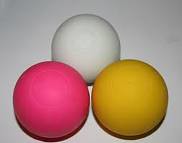In this small, closely-cropped, cube-shaped image, three perfectly smooth, round balls of matching size are meticulously arranged against a gray-to-white gradient backdrop. The background features darker gray in the top corners, transitioning to a lighter gray around the balls, giving a subtle, artistic contrast. Centrally placed at the top of the image is a slightly smaller white ball with a thin gray border. Directly below the white ball, almost forming a pyramid, are two larger balls: to the left, a vibrant, bright pink ball with a lighter pink circle on top, and to the right, a dull yellow ball. The balls are arranged such that the pink and yellow balls rest just slightly to the left and right of the white ball, creating a balanced and visually appealing symmetry. The smoothness of the balls and their striking colors set against the minimalist gradient background make for a captivating and harmonious visual composition.